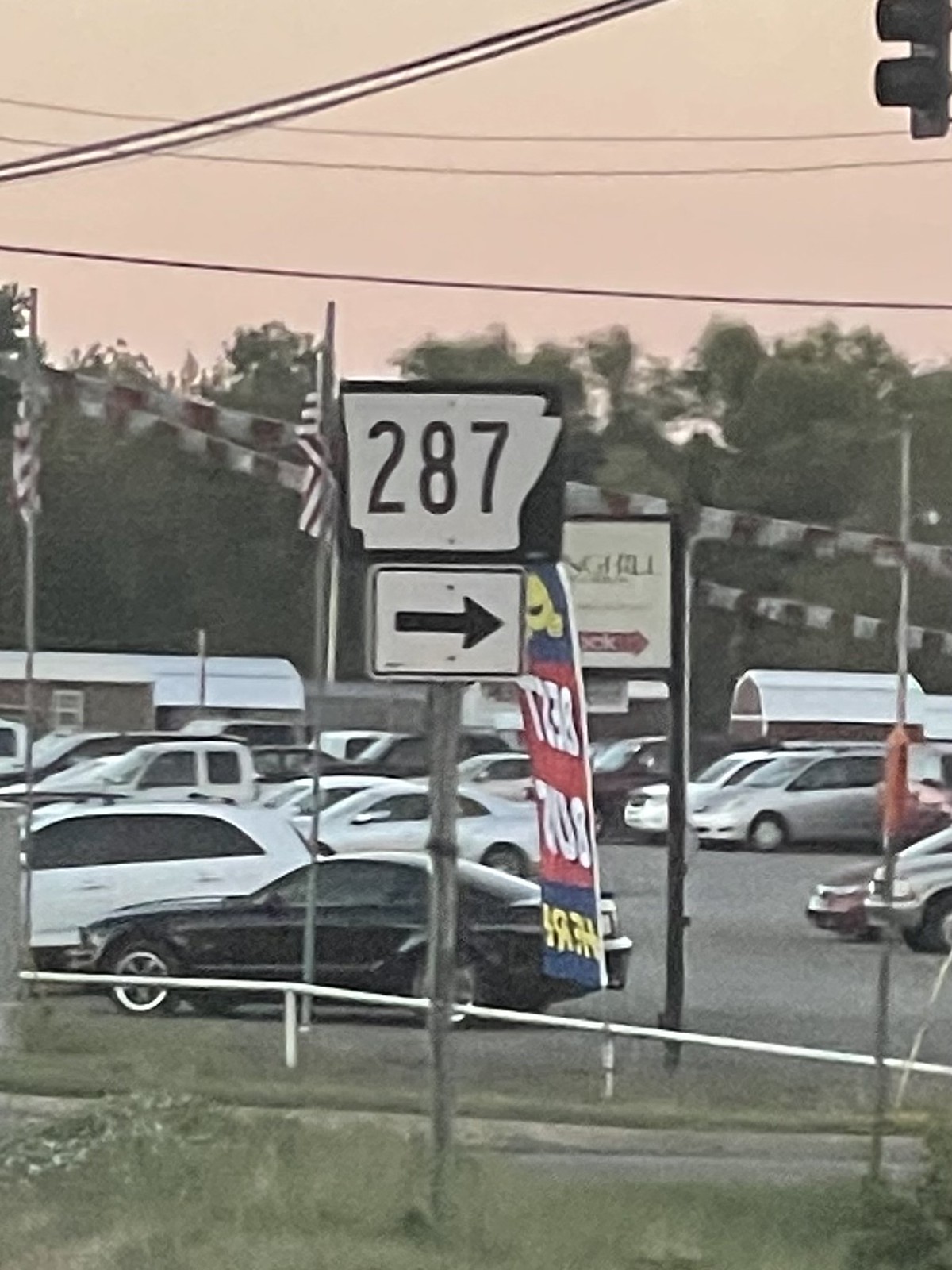The image captures an outdoor scene dominated by a street sign that reads "287" with a black arrow pointing to the right, mounted on a silver pole. In the background, a parking lot is filled with numerous cars, likely part of a dealership, indicated by a banner that reads "Best Buys here" in blue with gold or yellow writing. A large American flag flies prominently on the left side, accompanied by additional red and white banners strung across the lot, possibly connected by poles. The sky above has a light purple hue, dotted with electric wires and a street light in the top right corner. Surrounding the parking lot are lush green trees of varying heights, providing a verdant backdrop to the scene.